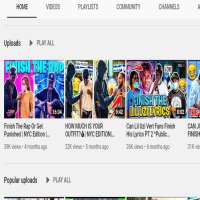The image depicts a small, hard-to-read, gray rectangle. At the top left corner, the word "Home" is visible, with a black bar below it. Next to this bar, there are four words written in gray, which are difficult to discern. Beneath this section lies another slightly darker gray rectangle with an arrow pointing to the right and text that appears to say "Upsides" or something similar, followed by more words that are unclear. Below this area are a series of small pictures that contain writing, possibly indicating they could be videos, but both the images and text are too small to read. Further down, there is additional text that is also too small to decipher. Towards the bottom, the phrase "Popular uploads" is barely readable, accompanied by an arrow pointing to the right and text that likely says "Play all." At the very bottom of the image, a colorful bar is present, featuring a pattern of colors including black, green, black again, green again, black, gray, and blue.